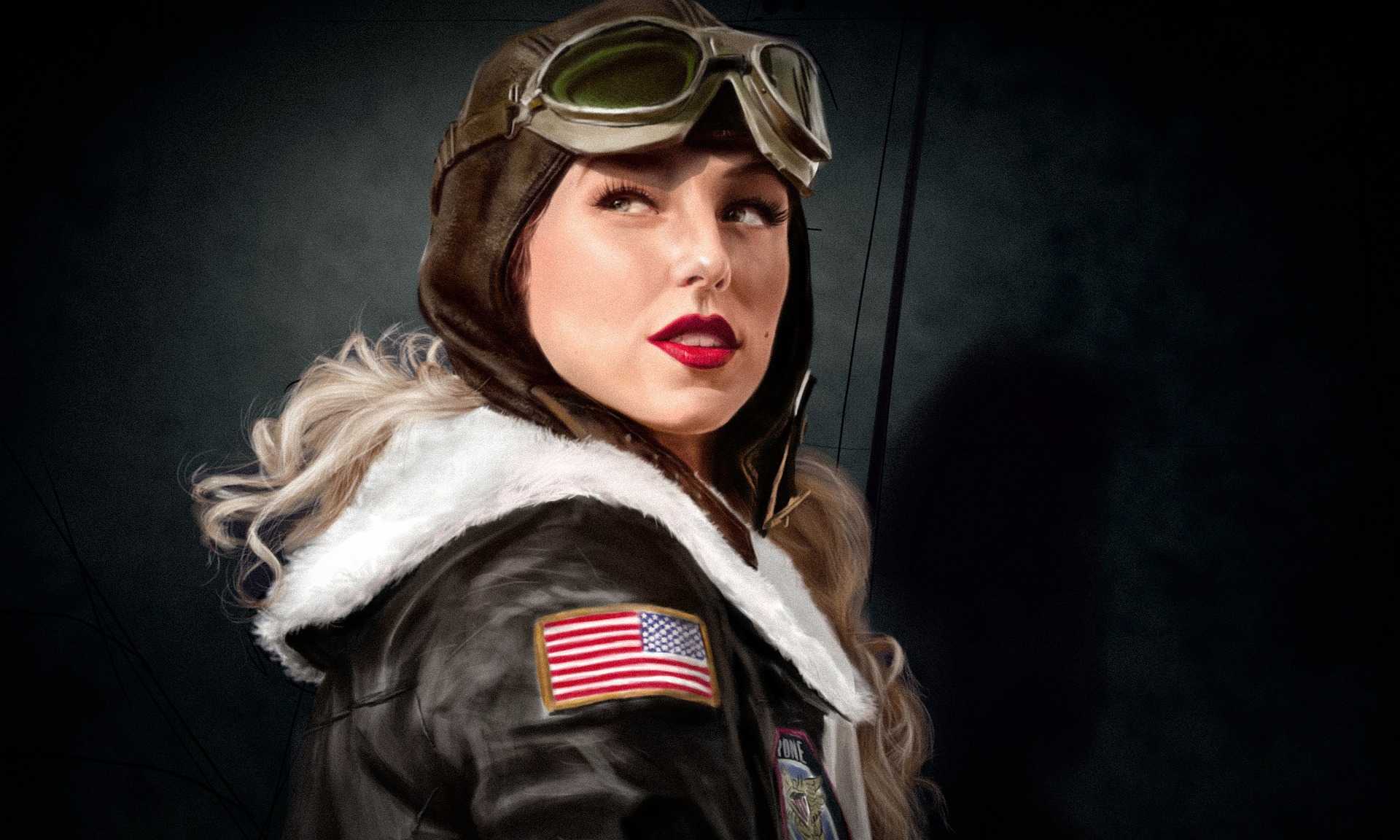This artwork depicts a woman strikingly resembling Taylor Swift, dressed as an aviator in the style of Amelia Earhart. She is positioned against a background of black and dark gray shades, enhancing the dramatic effect. The woman, with defining long blonde hair, sports a vintage brown leather aviator helmet adorned with goggles, which rest above her forehead. Her bright red lipstick contrasts vividly against her fair complexion. She is garbed in a leather bomber jacket with a distinct American flag patch on the shoulder, bordered in gold and featuring the classic red, white, and blue stripes. Her bomber jacket's exterior is brown leather while the inside fur lining is a contrasting white. As she gazes to her left with an introspective expression, her eyes look upwards, and a soft shadow is cast along the dark backdrop, adding depth to the scene.